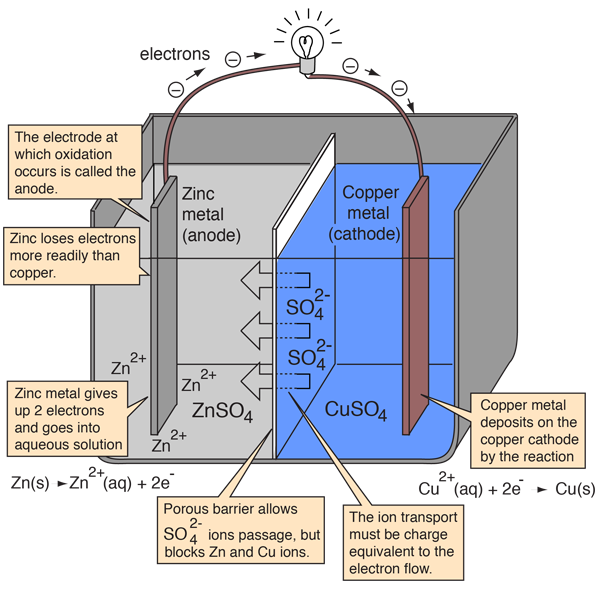This image is a detailed, colorful, technical infographic illustrating an electrochemical process, likely a battery operation. At the center, there is a cutaway tank housing two metal strips: the anode on the left, made of zinc, and the cathode on the right, made of copper. Connected to each electrode by copper-colored wires, a lit light bulb sits atop the diagram, with arrows indicating the flow of electrons from the zinc anode to the copper cathode. 

The backdrop features distinct colors: a light gray on the left side behind the zinc anode, and a blue on the right side behind the copper cathode. Surrounding the tank are several beige text boxes with black explanatory text and arrows pointing into the tank, detailing the processes and chemical reactions occurring within. In-tank black text includes specific chemical formulas like zinc sulfate and copper sulfate, with additional formulas provided on the lower left and right of the diagram, all set against a clean, white background.

The illustration not only highlights the materials and their roles but also visually demonstrates that the zinc anode undergoes oxidation by losing electrons more readily than the copper cathode. Black text at the top labels the flow of electrons, enhancing the educational value of this visually engaging technical chart.